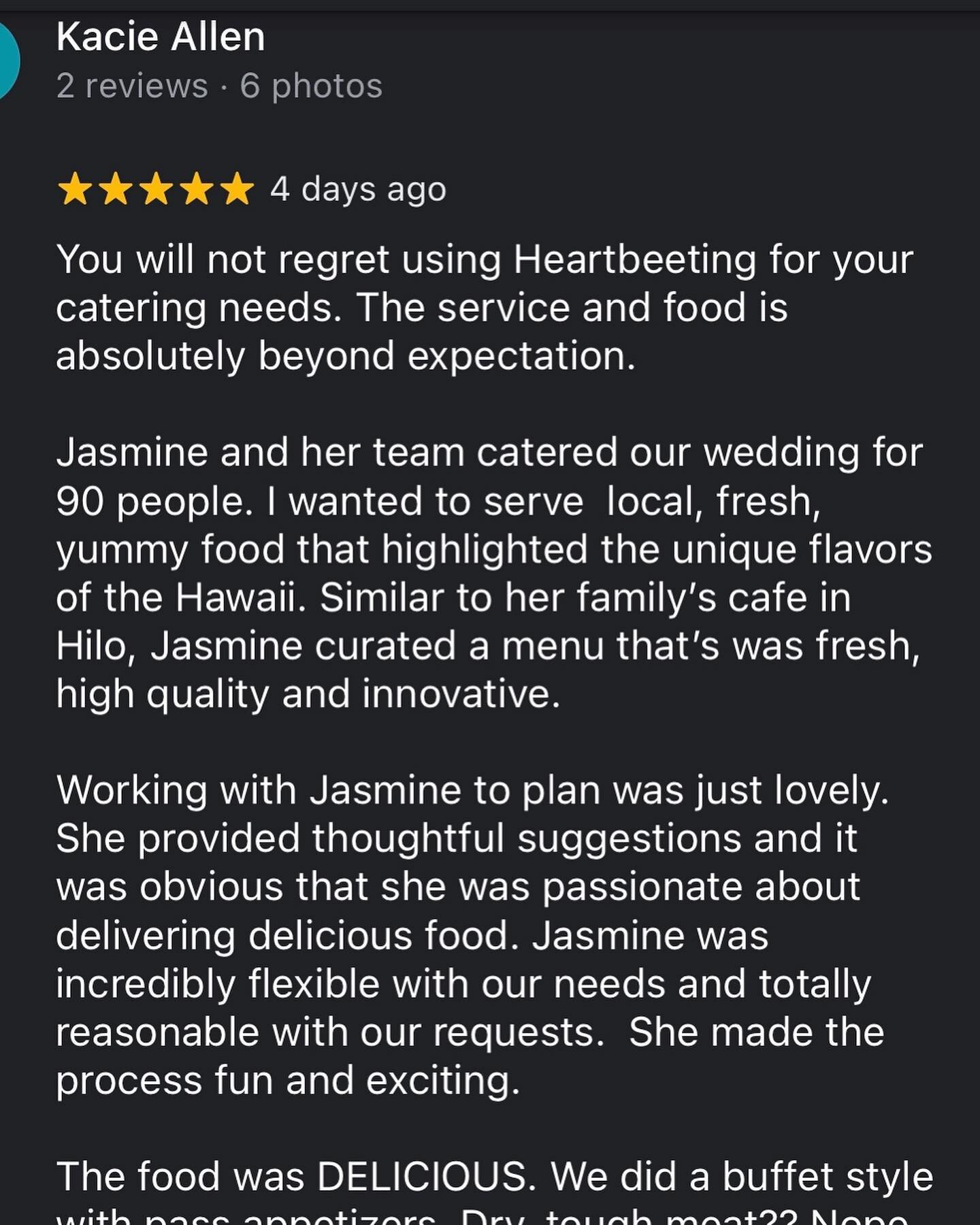Here is a cleaned-up and detailed caption for the image:

---

This image features a review by Casey Allen for Heartbeating Catering, accompanied by two additional reviews and six photos. Casey awarded Heartbeating a five-star rating four days ago. The review reads:

"You will not regret using Heartbeating for your catering needs. The service and food are absolutely beyond explanation. Jasmine and her team catered our wedding for 90 people, and we wanted to serve local, fresh, and delicious food that showcased the unique flavors of Hawaii, similar to her family's café in Hilo. Jasmine created a menu that was fresh, high quality, and innovative.

Working with Jasmine to plan was just lovely. She provided thoughtful suggestions and it was obvious that she was passionate about delivering delicious food. Jasmine was incredibly flexible with our needs and totally reasonable with our requests. She made the process fun and exciting. The food was delicious, served in a buffet style with passed appetizers. We couldn't have been happier with the catering."

---

This caption clearly conveys the details and sentiments expressed in the review, while removing any extraneous information.